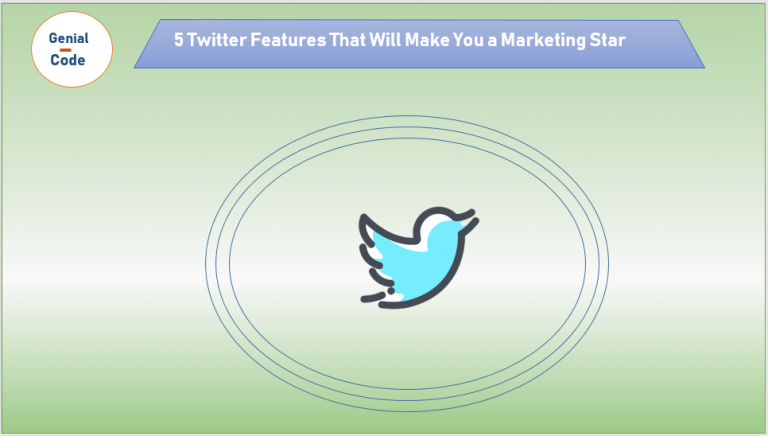The image features a rectangular, predominantly pale green background, with horizontal orientation. The background gradient transitions from a darker green at the bottom to a lighter shade in the center and then to a medium tone at the top. Central to the image is a stylized version of the Twitter bird, outlined in bold black with partial white coloring on its upper edges, deviating from the typical solid blue.

Surrounding the bird are three oval-shaped, gray lines that appear to be orbiting it. Above the bird, a narrow gray banner displays the text "Five Twitter Features That Will Make You a Marketing Star." This banner extends diagonally outward at the ends, giving it a flared appearance as it tapers towards the middle.

In the upper left corner of the image, there's a white circle outlined in gold. Inside this circle, the text "Genial Code" is written in dark green.